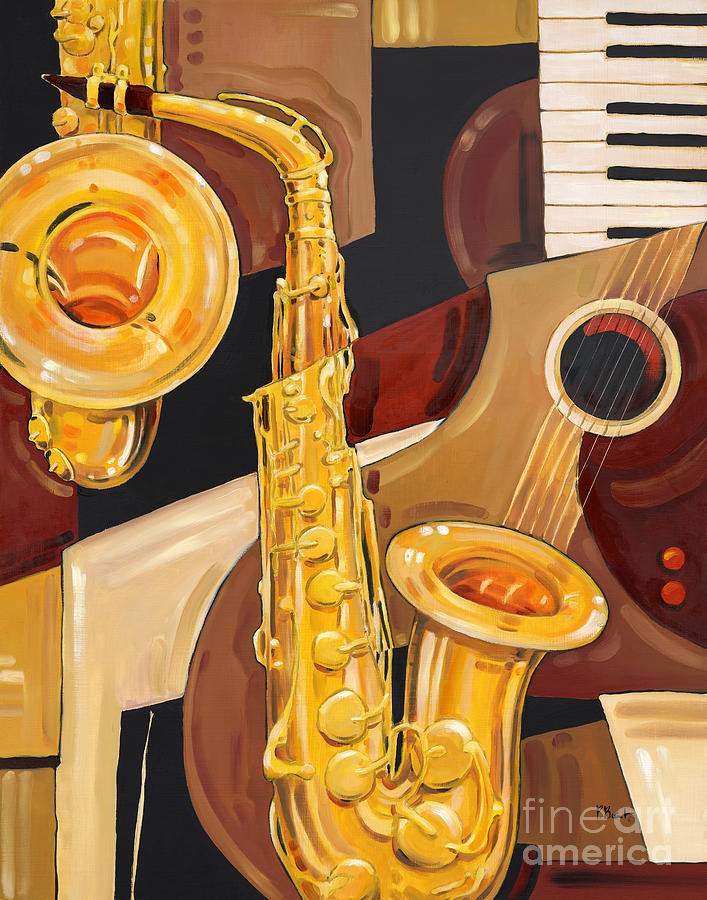The painting, likely associated with Fine Art America, features an assortment of musical instruments rendered in a stylized manner. Dominating the foreground is a yellow saxophone, which stands out prominently. To the top left, there appears to be another horn-like instrument, possibly another saxophone or a tuba, with a wide bell front. Accentuated in the top right corner are the black and white keys of a piano. Behind the central saxophone sits a guitar, characterized by its light tan body with darker elements and gold-tinted frets. The artwork uses a muted palette dominated by fall colors—yellows, browns, creams, golds, and ambers—with hints of black, white, and occasional red, giving it a warm, autumnal feel. Notably, the painting includes textual details: "Fine Art America" is elegantly inscribed in white at the bottom left corner.